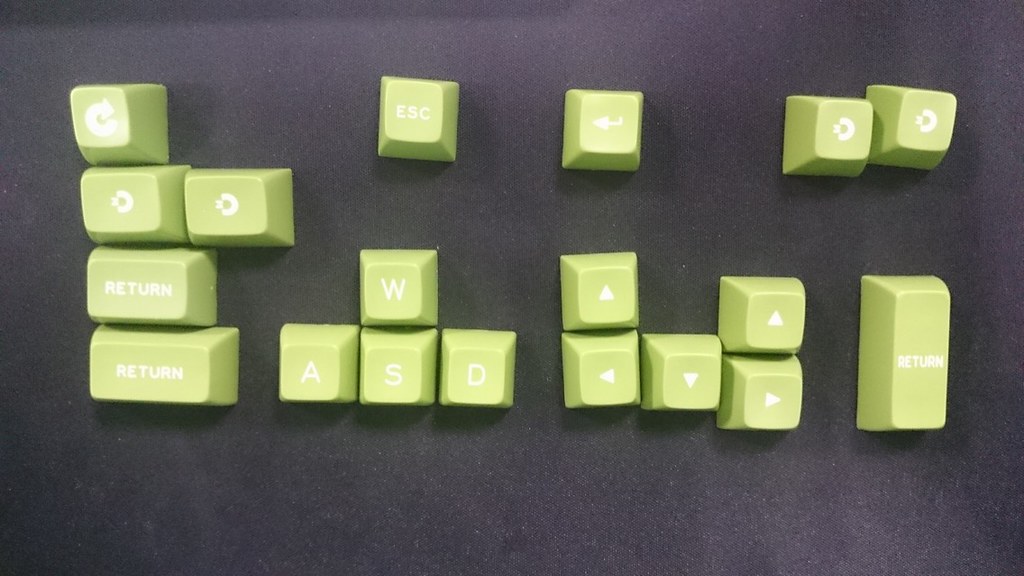The image showcases various lime green keyboard keys with white letters and symbols, scattered across a smooth black surface, possibly a tabletop or floor. On the left side, there are four keys arranged in a vertical column, with the bottom two marked as "Return" keys, the lower ones being larger. To the right of this column, there are three square keys labeled "A," "S," and "D," with a "W" key positioned above the "S." Adjacent to these are three arrow keys indicating left, right, and down directions, and a rectangular vertical key also labeled "Return." Spread across the top of the image are several other keys, including an "Escape" key, five arrow keys pointing in different directions (two facing upwards), two keys with stylized "D" logos, and a key with a circular arrow symbol. Some keys appear to have white dots in their centers, adding to the peculiar arrangement of these detached keyboard buttons.